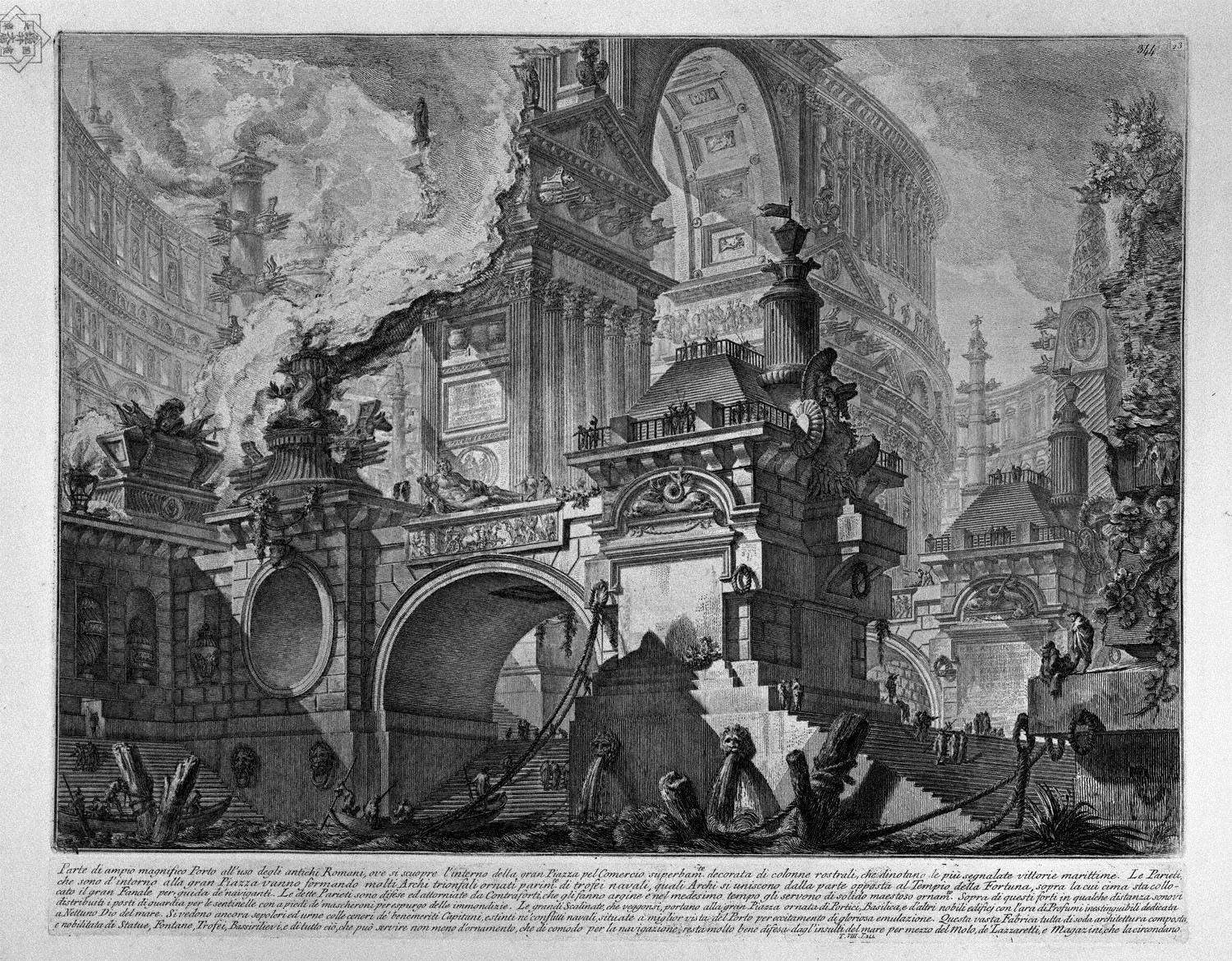This black and white pencil drawing is an intricate and elaborate depiction of a partially destroyed cityscape, reminiscent of Roman architecture. Central to the composition is a grand, stately structure echoing the form of the Roman Colosseum, with sweeping arches and impressive columns. The building, which also evokes the majesty of the Arc de Triomphe, appears war-torn, with sections missing and smoke billowing from the upper left corner. On the right-hand side, a clock tower stands prominently, surrounded by carved statues and what seems to be a fountain with a lion's face spouting water. The foreground is littered with debris, bricks, and shattered columns, adding to the scene's sense of ruin and chaos. The sky is depicted with wavy, tumultuous shapes, enhancing the overall impression of destruction. Below the illustration, a lengthy paragraph of text in English seems to provide context or explanation for the scene.